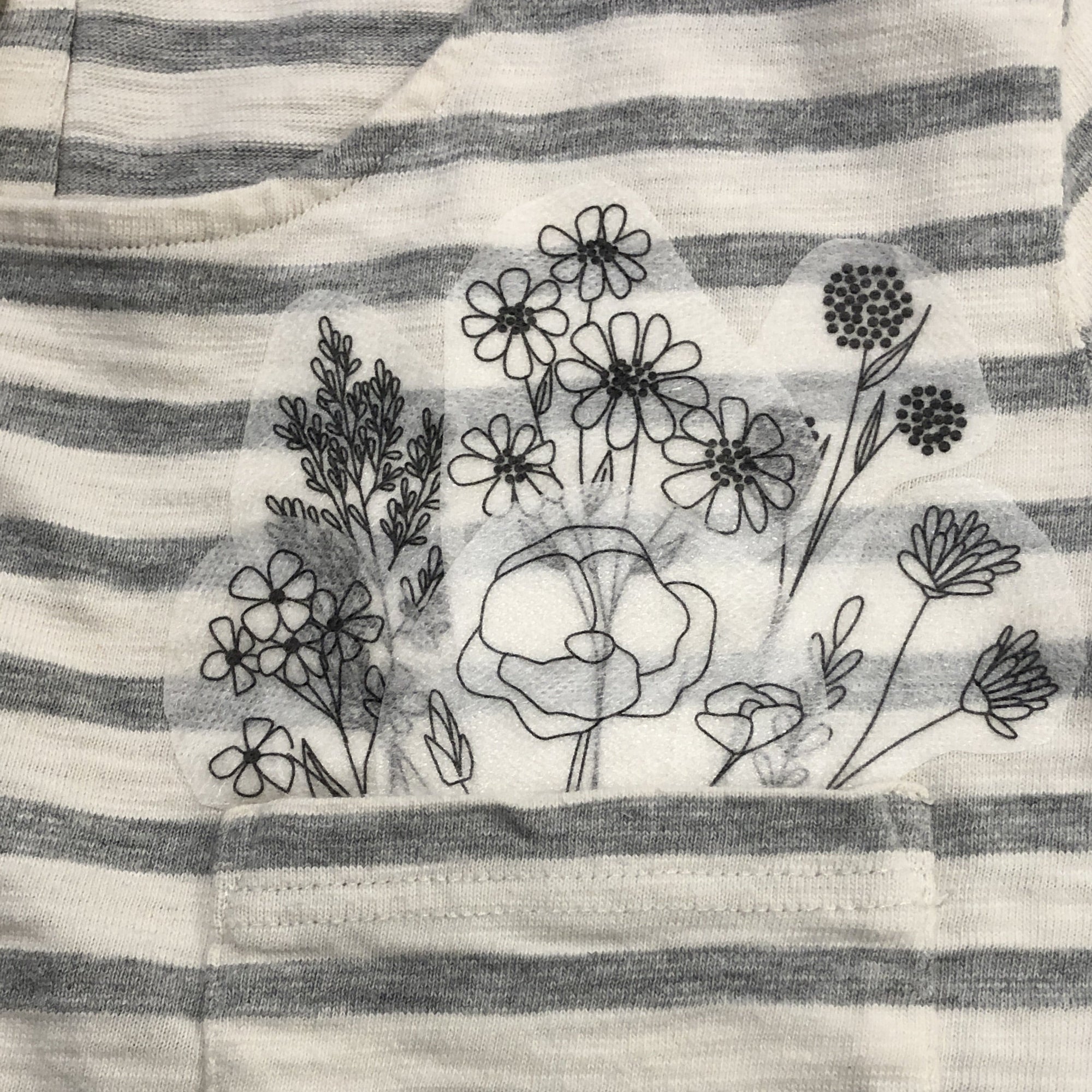The image showcases a close-up of a women's short-sleeve shirt made of thin white cotton fabric, interspersed with horizontal gray stripes. It features a matching striped pocket located on the chest area, which is accentuated by intricate black outline stitching. This stitching forms an arrangement of flowers and leaves, all detailed in a sketchy, monochromatic style on interfacing-type non-woven fabric pieces, possibly iron-on patches. The floral designs—ranging from daisies and carnations to generic flowers and small leafy branches—vary in size and detail. Notably, some of these floral pieces appear positioned as if tucked or arranged within the pocket. The shirt is designed with a delicate, rounded crew neckline, enhancing its feminine appeal.